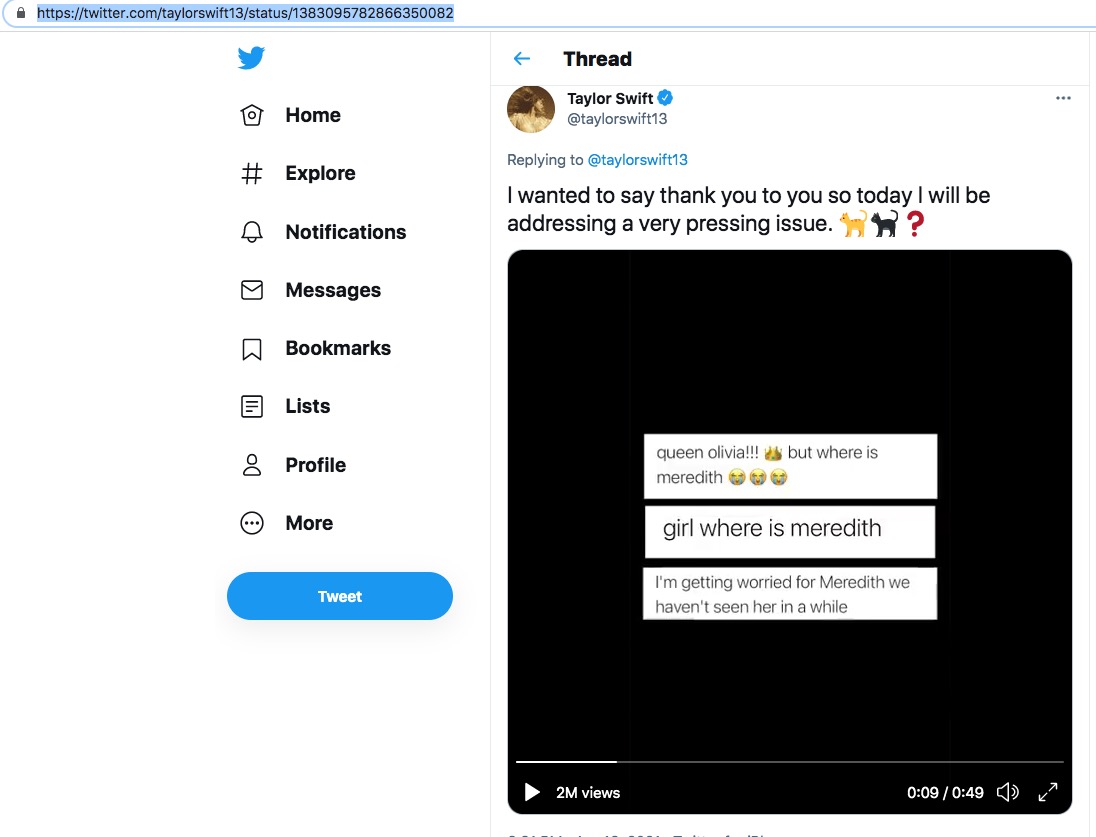This is a screenshot of a Twitter feed, featuring a navigation bar at the top with indistinct edges, which seamlessly blend into the rest of the page. Directly below, there's the typical sidebar menu from Twitter (or X), showcasing familiar icons: the blue bird for Home, a birdhouse icon, a hashtag for Explore, a bell for Notifications, and icons for Messages and Bookmarks. 

In the center of the screenshot is a tweet from Taylor Swift, which reads, "I wanted to say thank you, so today I will be addressing a very pressing issue." The post includes a few cat emojis and a question mark. The attached image within Taylor Swift's tweet features a black background with screen-capped tweets from fans. One of the tweets reads, "This is Queen Olivia, but where's Meredith girl? Where is Meredith? I'm getting worried for Meredith; we haven't seen her in a while." There appears to be a video included as part of the post, though its content is not clear from the screenshot. 

The screenshot likely captures a moment of fan interaction regarding Taylor Swift's pets, with particular concern about a lack of recent appearances from her cat, Meredith.